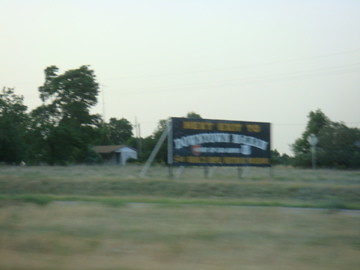An overcast sky sets a somber mood in this scene captured along a highway. A line of trees and various distant buildings, along with some utility poles and a tall antenna to the right of the tallest tree, stretch across the horizon. However, the center of attention is a large, out-of-focus billboard. Despite the blurriness, the words "Next Exit" and "Downtown" can be discerned, while the rest of the text fades into unreadable smudges, potentially hinting at a museum. The billboard, supported by four posts with an additional support post at the back, stands resiliently over a grassy pasture in the foreground. The overall distortion of the image suggests it was taken from a rapidly moving vehicle, resulting in the captured motion blur.